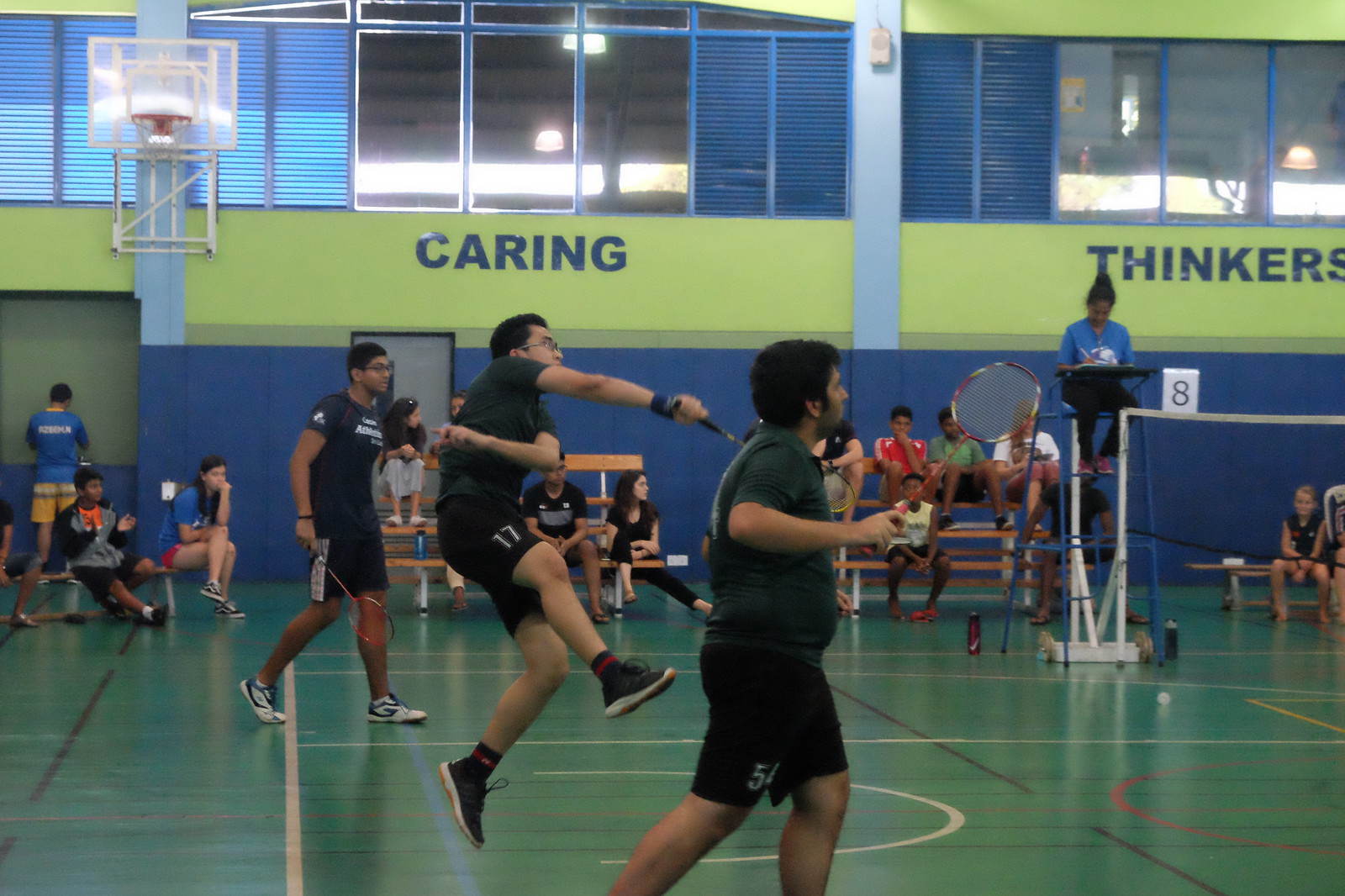The photograph captures an indoor badminton game in a multi-use gymnasium. In the center foreground, there are three players actively engaged in a match, each wielding a badminton racket. One player, positioned on the left, has just made a hit, sending the shuttlecock towards the opponent's side. Another individual stands on a step ladder stool next to the white badminton net, presumably serving as a referee or official overseeing the game. The court itself is a dark green color, marked with various white, black, and red lines indicating different areas of play.

The gym's far back wall, predominantly visible in the image, is covered with thick blue pads at the bottom for protection. Above the pads, the wall is painted lime green and features blue text with the words "caring" and "thinkers." Scattered blue support beams segment the wall, adding structural detail. Higher up, multiple windows with blue frames and matching blue window blinds let in natural light, accentuating the vibrant color scheme.

In the background, a group of people can be seen seated, possibly on a set of bleachers or individual chairs, watching the game. Additionally, a basketball hoop hangs in the top left corner, indicating the gym's multifunctional use for various sports. The entire setting reflects a lively atmosphere of recreational activity and sportsmanship.